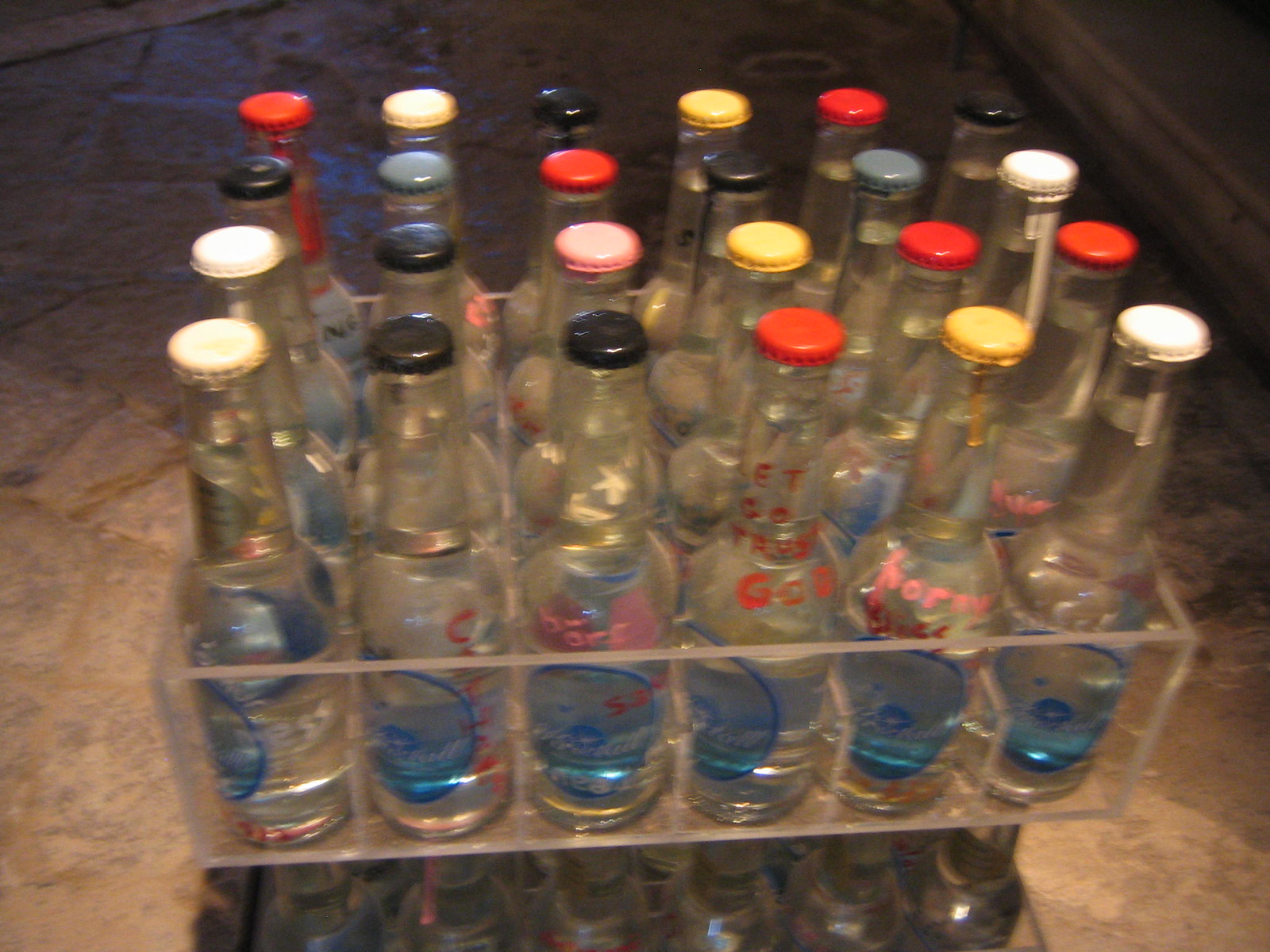This fuzzy horizontal rectangular photograph depicts 24 clear glass bottles, each capped with various colors, arranged in four rows of six within a clear plastic crate with dividers. The crates, which appear to be acrylic holders, are stacked—one centered and visible, and another underneath partially visible. The bottle caps come in different colors: white, black, red, blue, pink, gray, orange, and yellow. The clear bottles, which may contain either a clear liquid or nothing inside, feature blue oval labels, outlined in medium-toned blue, with possible black-eyed and black-nosed animal faces. Some bottles also display hand-lettered text in red, pink, or white. The text is partially legible, with fragments like "ET CO TA" visible on one bottle. The entire setup rests on a tan floor, with light brown stone-like tiles. Additionally, part of a wall molding is seen in the upper right corner of the frame.